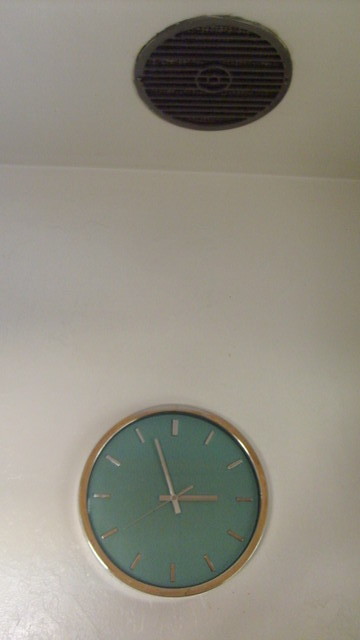This vertically oriented photograph captures an analog clock mounted on a white wall, positioned in the lower third of the image. The clock features a gold metal frame and a desaturated teal face, contributing to its minimalistic design. Instead of numbers, the clock face displays dashed lines, with bolder marks at the 12, 1, 2, and 3 o'clock positions. It shows the time as 2:57, with the second hand nearly touching the 8. The clock's hands are gold or potentially silver. Above the clock, the photograph captures the intersection where the ceiling meets the wall. On the ceiling, there is a round, black recessed element with horizontal slots that might function as a speaker, air conditioning vent, or smoke detector.